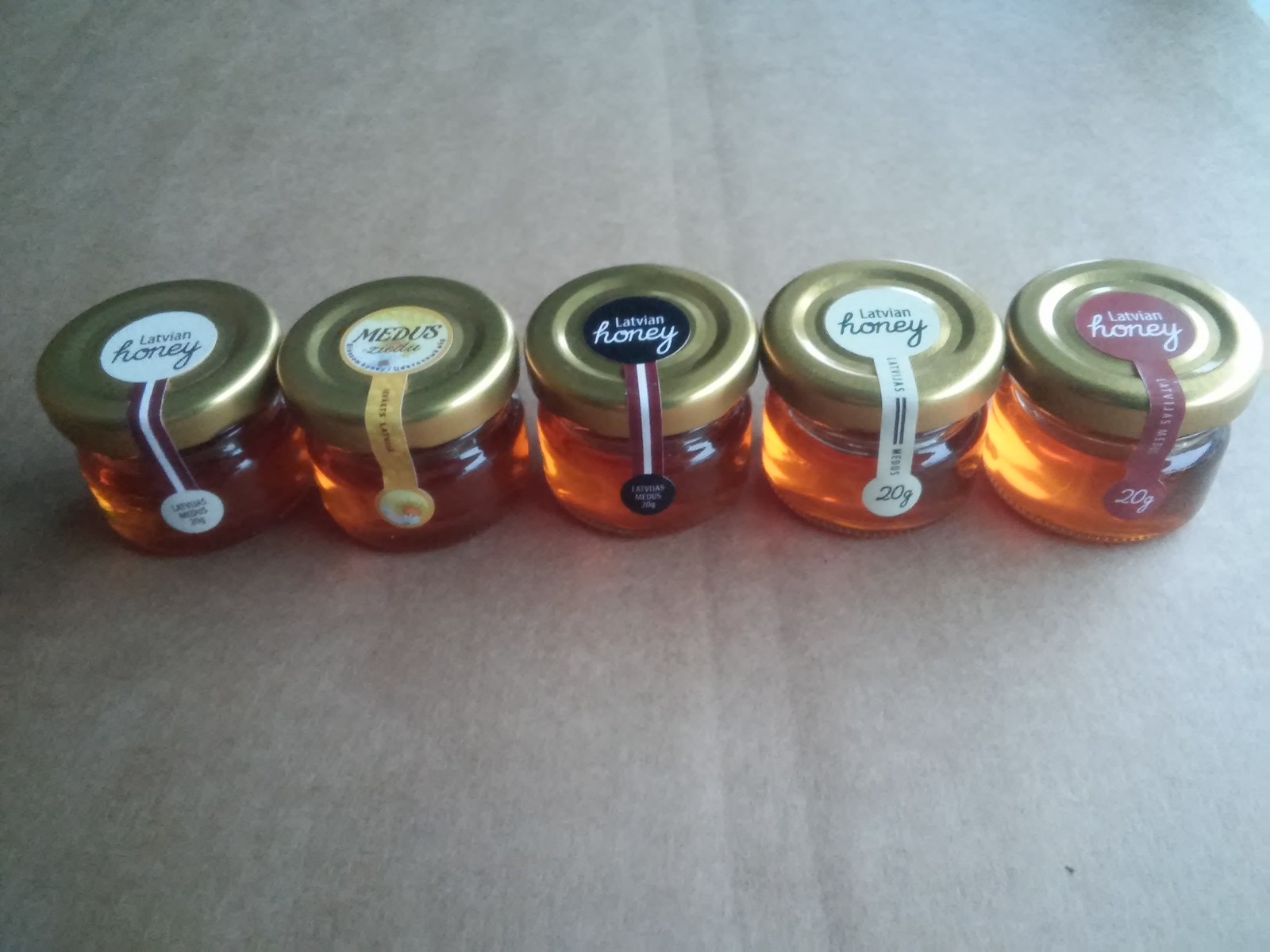The photograph displays five small jars of honey, neatly arranged in a horizontal line on a light-colored fabric. Each jar, made of clear glass, reveals the golden honey inside. They are capped with circular, twist-off golden lids. At the center of each cap, there is a small, circular label. The leftmost label is white with black text reading "Latvian honey." The second label is yellow and white, inscribed with "medus" or "medas." The middle jar features a black label with white lettering stating "Latvian honey." The fourth jar returns to a white label with "Latvian honey" in black font, while the final jar has a red label also reading "Latvian honey" in white text. Each cap has an elongated rectangular sticker that runs from the top down the side of the jar, acting as a seal that breaks when the lid is first twisted off. The honey jars, each holding 20 grams, are uniform in shape, resembling small lotion bottles. They are set on what appears to be a brown surface, providing a contrasting backdrop to the light fabric.